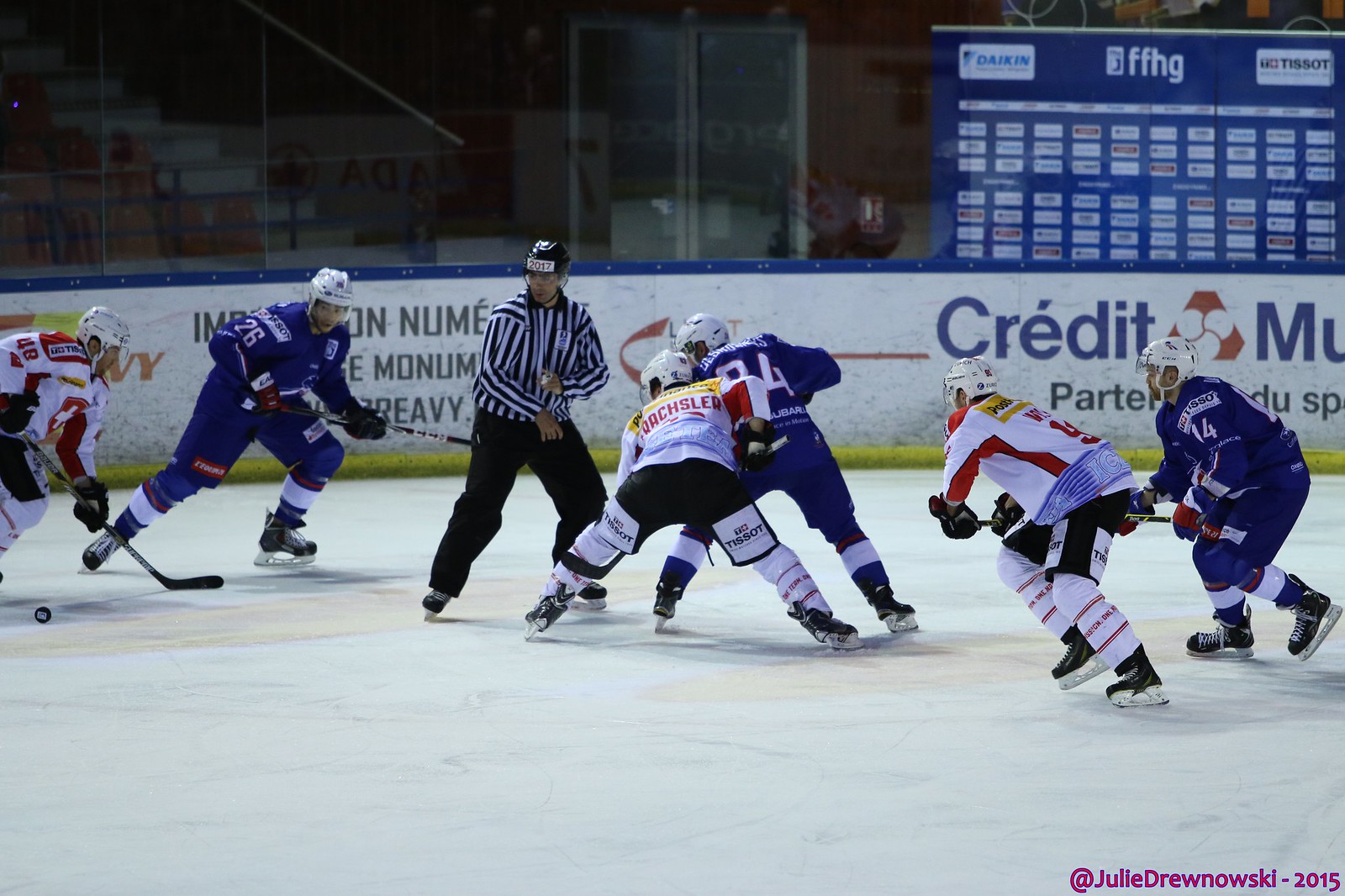This detailed action shot captures an intense moment during an indoor ice hockey game. The two competing teams are dressed in distinct uniforms; one team in blue jerseys and white helmets, and the other in white jerseys with red accents, complemented by black shorts and white padding. Both teams are gripping their hockey sticks and racing toward each other across the ice. Centrally positioned is a referee in a black and white striped shirt and black helmet, actively monitoring the play.

The background features a shaded seating area with bleachers, their occupancy unclear due to the shadow. Surrounding the rink, billboards display various sponsors, including names like Credit, Amu, Partner, NUMI, Monam, and RIVI. Additional banners with logos such as Daikin, FFHG, and T-Short are visible at the top right corner.

On the right side of the image is a blue scoreboard with multiple boxes, though its details are not readable. Noteworthy is the bottom right-hand corner of the image, which features the inscription "© Julie Drewnowski - 2015."